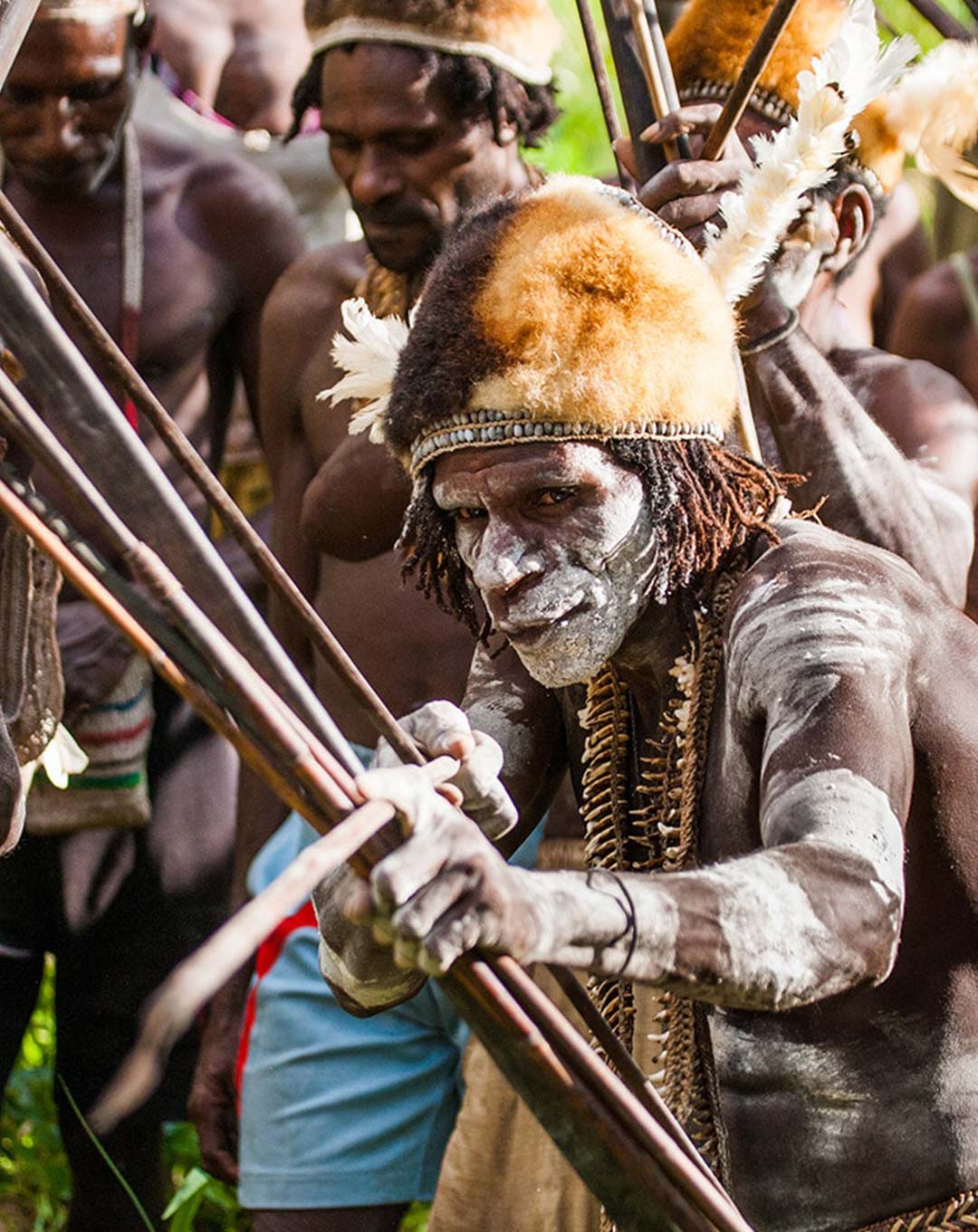This outdoor photograph captures a close-up of Azmat warriors from New Guinea, set against a grassy field. Dominating the bottom right of the image is an older man with dark brown skin, his body turned left while his head is tilted closer to the camera. His skin is adorned with white paint, which forms stripes down his arms and covers his shoulders, nose, and cheeks. His face is framed by black and brown thin dreadlocks, partially covered by a distinctive fuzzy hat, orange on one side and black on the other. The hat appears to be made from animal hide with feathers sticking out.

He grips a wooden bow and arrow with both hands, the arrow poised to shoot towards the lower left of the frame. Around his neck, he wears a traditional beaded necklace. Behind him, several shirtless men, seemingly of the same tribe, share similar skin tones and sport identical headgear and necklaces. They form a line, each holding a bow and arrow, signifying their unity and shared cultural heritage. The overall scene, with its detailed depiction of tribal attire and weaponry, offers a vivid portrayal of these Azmat warriors.